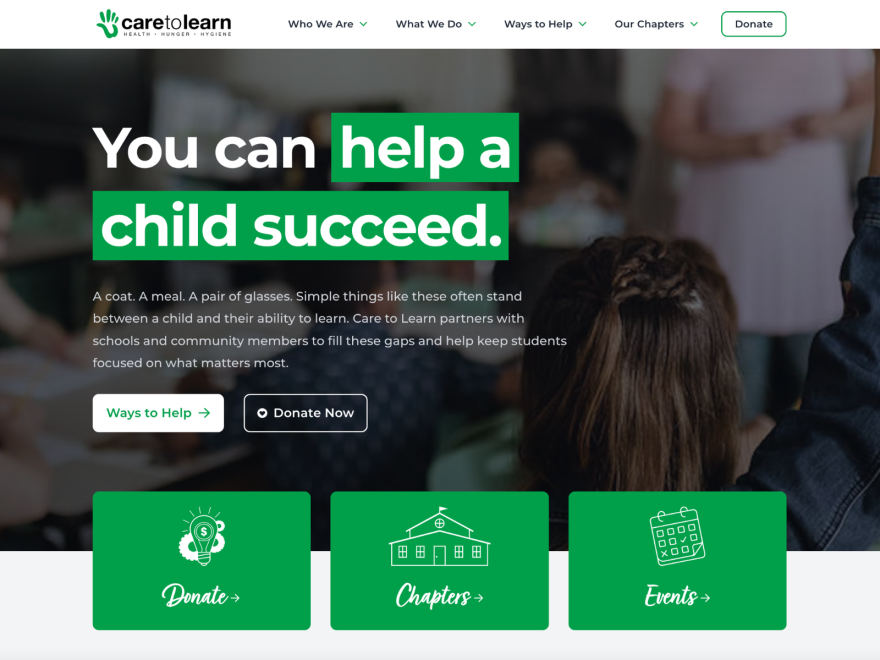The image appears to be a promotional graphic for an organization dedicated to assisting children by addressing basic needs crucial for their education. The top of the image features a bolded phrase "care to learn," written in all lowercase letters. Underneath, in smaller text, it lists the core areas the organization focuses on: health, hunger, and hygiene. To the left, there is a green hand symbol.

To the right, sections titled "Who We Are," "What We Do," "Ways to Help," and "Our Chapters" provide more detailed information or categories for further exploration. There's a prominent "Donate" button nearby.

Beneath these sections, a photograph depicts students engaged in learning, with their backs turned to the camera. Overlaying the photo is the text "You can help a child succeed," with the phrase "help a child succeed" highlighted in green.

Further down, a smaller white text reads: "A coat, a meal, a pair of glasses, simple things like these often stand between a child and their ability to learn. Care to Learn partners with schools and community members to fill these gaps and help students focus on what matters most."

At the bottom, there are two buttons: "Ways to Help" and "Donate Now." Additionally, three green boxes offer further actions: the first for "Donating," represented by a money symbol and a flashbulb or light; the second for "Chapters," symbolized by a building icon; and the third for "Events," marked by a calendar icon.